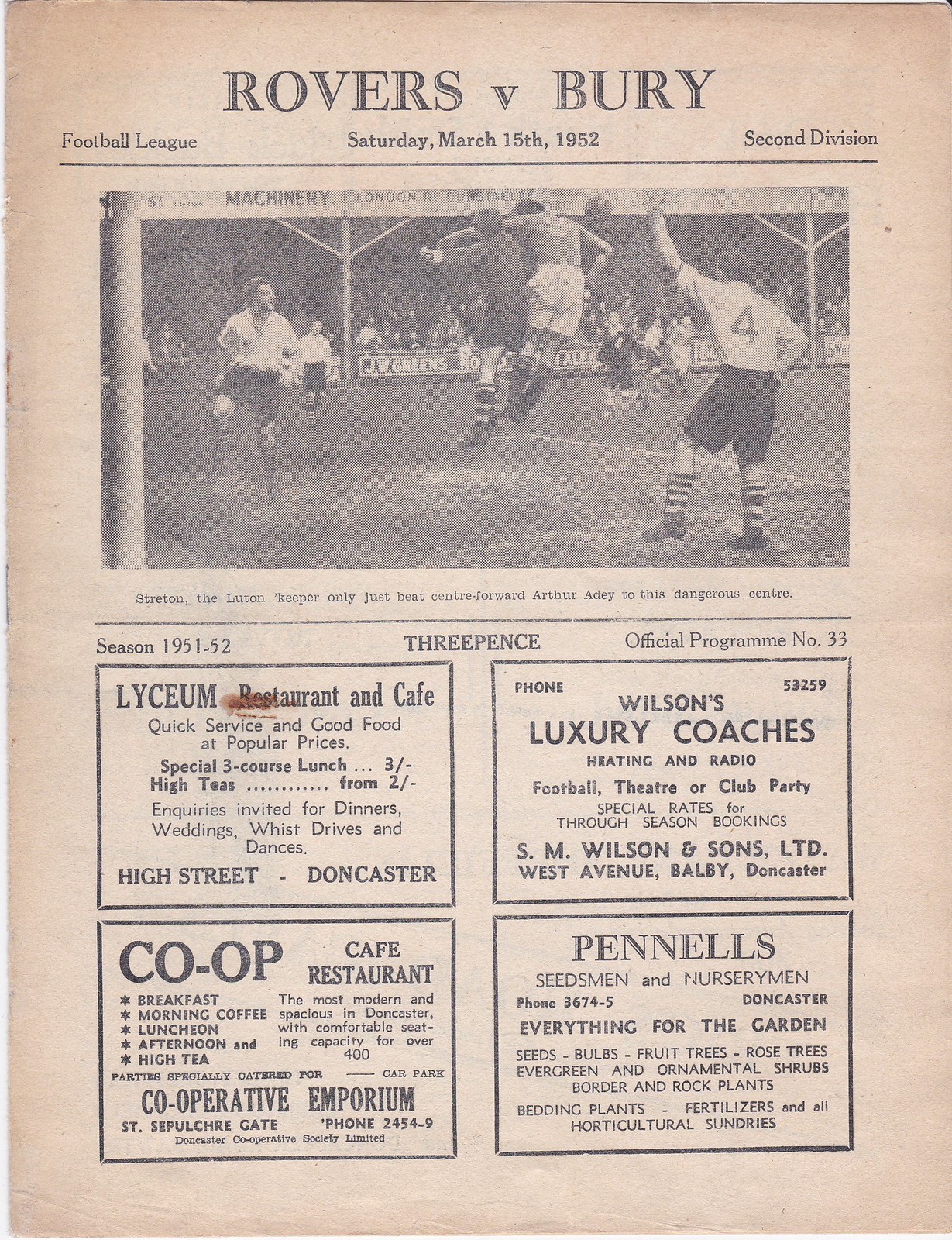This image is a detailed and vintage black-and-white printed cover of a program for a football league match between Rovers and Bury, held on Saturday, March 15, 1952, in the 2nd Division. The program is printed on aged paper in portrait orientation, with a stark black headline that reads "Rovers vs. Bury" at the top, flanked by smaller text specifying "Football League" on the left, the date in the center, and "2nd Division" on the right. Below this information, a horizontal line separates the header from a landscape-oriented black-and-white photograph that captures an intense moment of gameplay: several young football players in uniform are seen jumping and playing, with fans visible in the background. The photograph's caption reads, "Streaton, the Luton keeper, only just beat center forward Arthur Eaddy to this dangerous center." The bottom half of the page displays four rectangular advertisements arranged in two rows of two, promoting local businesses such as the Lyceum Restaurant and Cafe, Wilson's Luxury Coaches, Co-op Cafe Restaurant, and Pinnell's Seedsmen and Nurserymen. Above these ads is a line that states, "Season 1951-52," with the price "3 pence" and "official program number 33" positioned to the right. The entire style of the program is distinctly vintage, echoing the print publication aesthetics of the early 1950s.